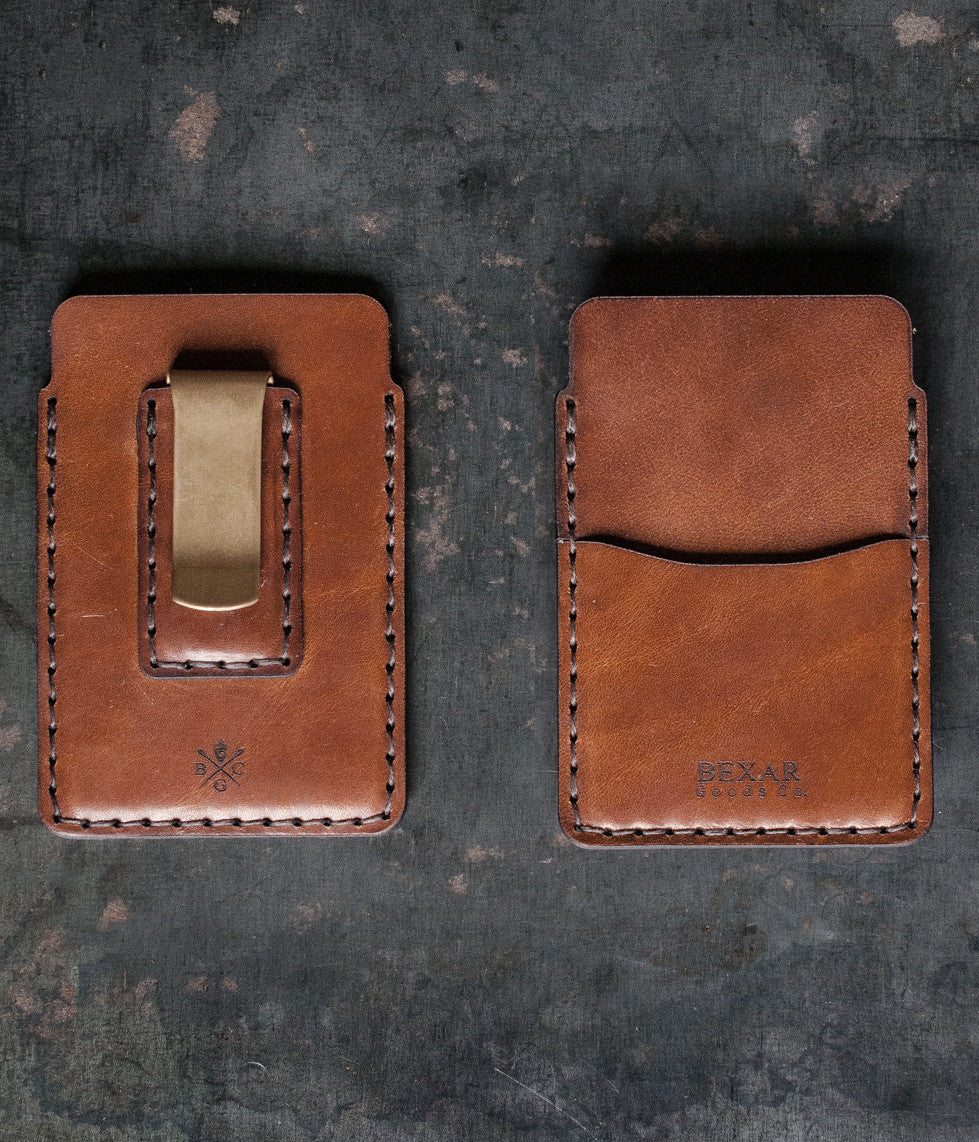This is a large interior photograph of two brown leather money clips or card holders resting on a rugged, gray, metallic surface with natural white splotches. The objects are small and square, intricately sewn with thick black stitching around the edges and bottom. Each object has distinctive features; on the left, there is a brass-colored clip attached to its back, designed to clip onto a belt or pocket, while the one on the right features a pouch capable of holding items like credit cards. Both have graphical branding; the left clip's bottom showcases an X logo with the letters B, G, and C in each segment, and the right clip features the embossed name "Bexar Goods Company" at the bottom, though the low contrast makes it somewhat hard to read.